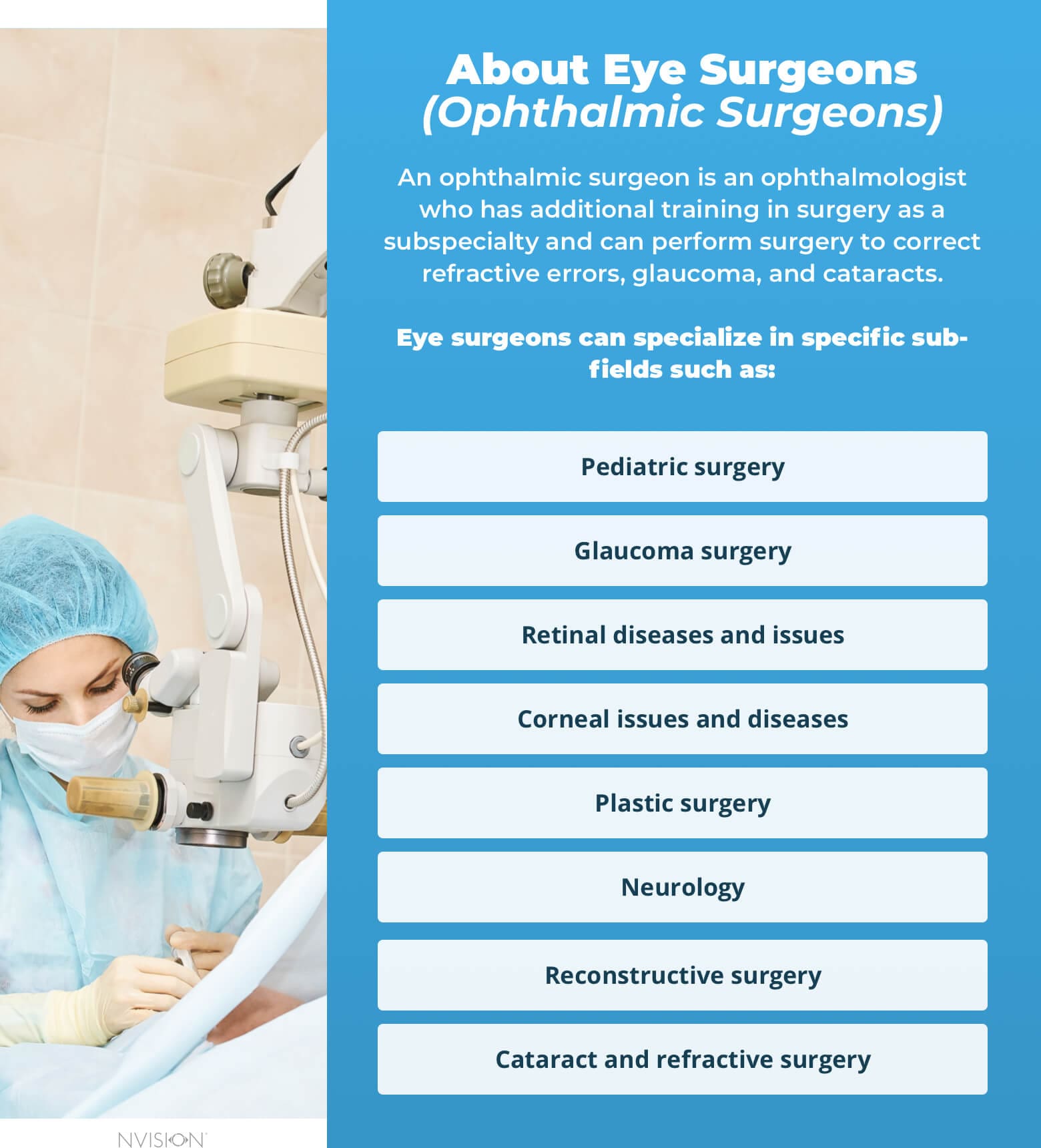The poster presents information about ophthalmic surgeons, also known as eye surgeons. It's divided into two main sections: the left side features an image, while the right side contains detailed text. 

On the left, a woman is dressed in blue scrubs, complemented by a white face mask, a blue hairnet, and white gloves. She stands in front of a large piece of medical machinery, possibly an imaging or x-ray machine, engaged in an activity with her hands. 

The right side of the poster has an informational section with a blue background. The top section, titled "About Eye Surgeons" with "ophthalmic surgeons" in parentheses, explains that these are ophthalmologists who have additional surgical training. The text elaborates on their ability to perform surgeries to correct refractive errors, glaucoma, and cataracts. Further down, the poster lists specific sub-fields in which eye surgeons can specialize: pediatric surgery, glaucoma surgery, retinal diseases and issues, corneal issues and diseases, plastic surgery, neurology, reconstructive surgery, and cataract and refractive surgery. The bottom of the poster features the text "NVISION" in black print, indicating the name or branding of the organization behind the poster.